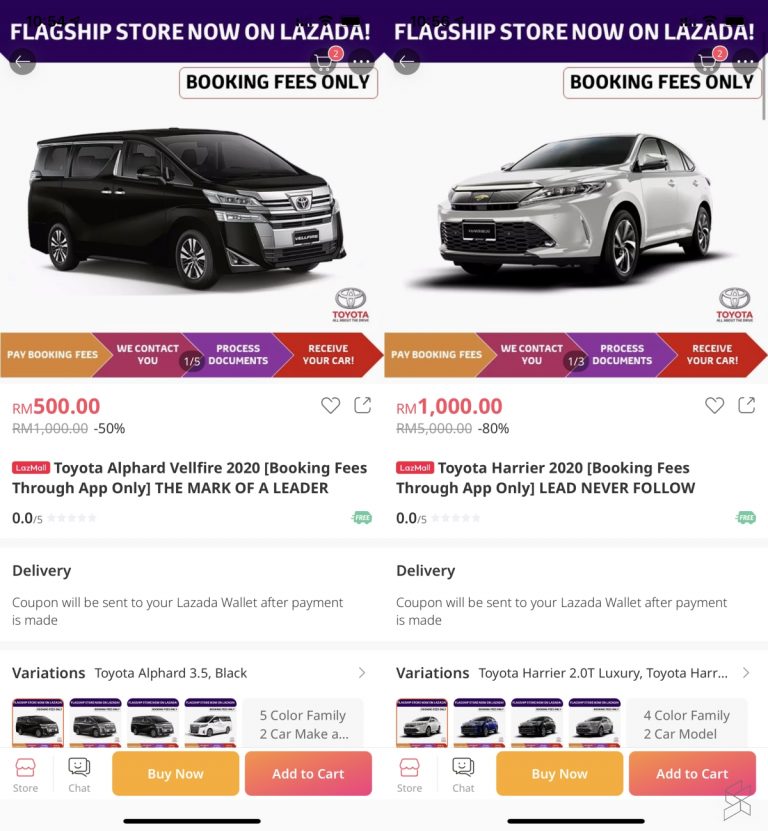This detailed caption describes a complex screenshot taken from a cell phone, displaying a dual-column layout in portrait mode. The screenshot showcases an online shopping platform, possibly Lazada, with two different car purchase options. 

### Left Column:
- **Header:** A large purple banner with partially visible text that appears to say "Flagship Store Now on Lazada."
- **Navigation Bar:** Includes a back arrow, a shopping cart with two items, and an icon featuring three dots in a circle.
- **Button:** A rounded rectangle button that might say "Booking Fees Only."
- **Product Image:** A large image of a Toyota SUV.
- **Step-by-Step Instructions:** "Pay booking fees, we contact you, process documents, receive your car."
- **Carousel Indicator:** "1 of 5," hinting at multiple images or steps.
- **Purchase Details:** "RM 500, minus 50%."
- **Product Information:** "Laz Mall Toyota Alphard Vellfire 2020, Booking fees through app only, The mark of a leader."
- **Delivery Info:** "Delivery coupon will be sent to your Lazada wallet after payment is made."
- **Variations:** Options for different choices related to the product.

### Right Column:
- **Header:** The same large purple banner as in the left column.
- **Product Image:** This time showing a different car, the Toyota Harrier 2020.
- **Product Slogan:** "Lead Never Follow."
- **Purchase Details:** "RM 1000, minus 80%."
- **Variations:** Options for different choices related to this model as well.

The overall image captures the side-by-side comparison of two Toyota models available for online purchase through a shopping website, emphasizing convenience, discounts, and additional options for customization.